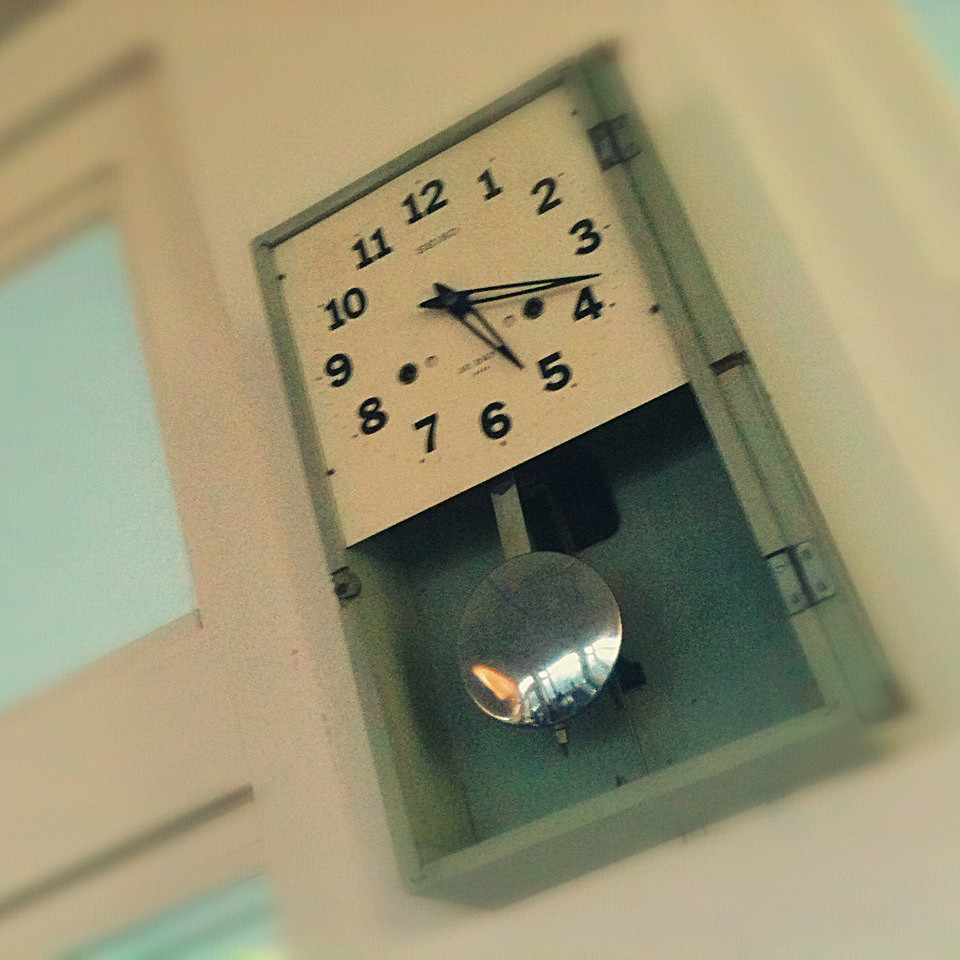This detailed photo captures a close-up of a rectangular wooden clock mounted vertically on a predominantly white wall. The clock face, situated in the top half of the rectangle, is white with black Arabic numerals and includes black hour and minute hands, along with a second hand. It displays the time as approximately 5:18. The clock is protected by a cover secured with clamps. Below the clock face, a metal pendulum with a round end swings from side to side, adding to the clock's vintage appearance. The setting suggests an older institutional building, such as a school or clinic, distinguished by the simplicity and utilitarian design of the clock. The background reveals a turquoise section in the upper right corner and another turquoise section at the bottom left of the image. To the left of the clock, there is a door featuring a turquoise window at the top, adding a splash of color to the otherwise stark white environment. Overall, the scene evokes a sense of nostalgia and practicality.